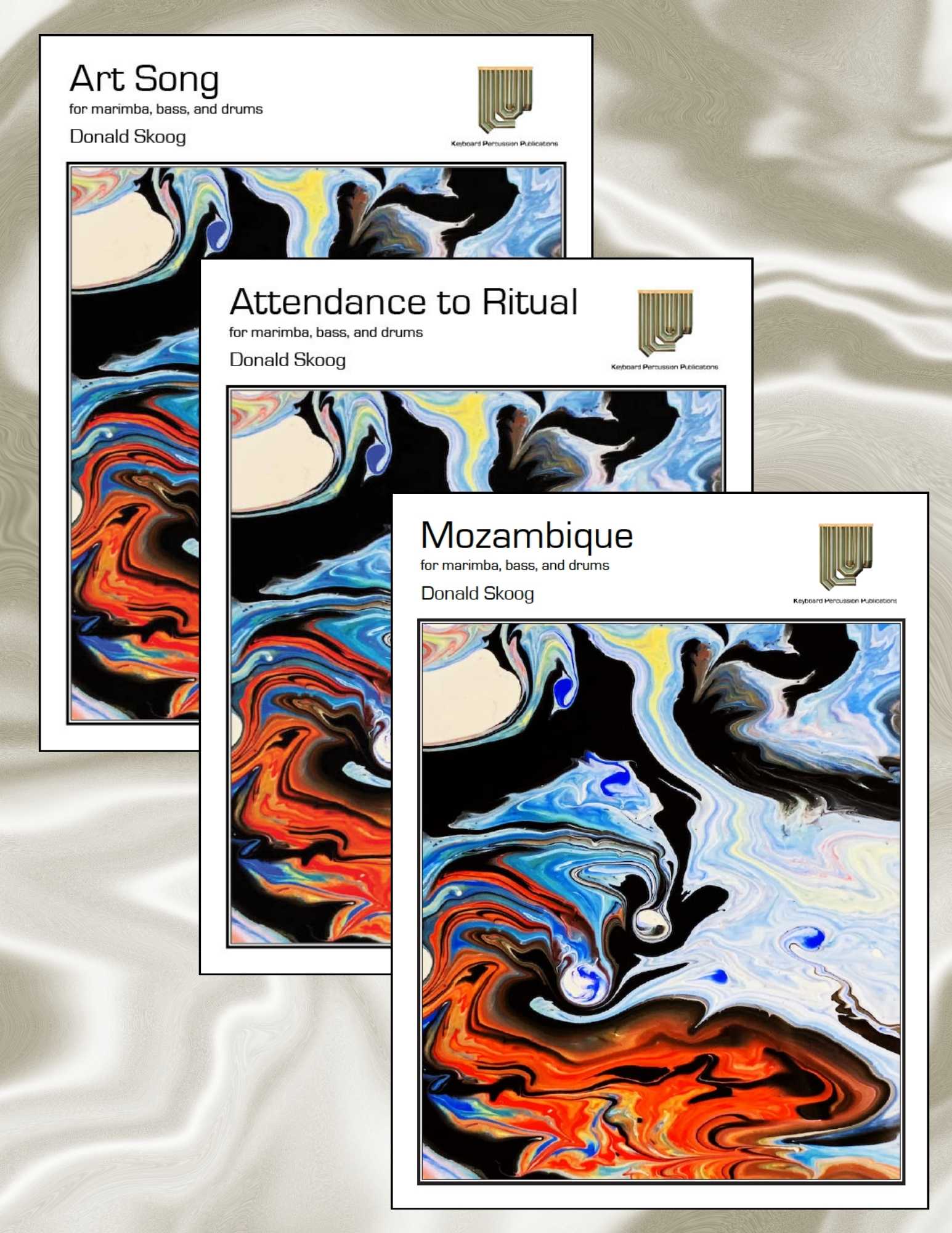The image depicts three rectangular illustrations, slightly overlapping each other, set against a background that appears to be white satin. Each illustration features an identical abstract design reminiscent of swirling oil on water, incorporating colors like black, orange, dark blue, along with lighter pastel shades. These artistic visuals contain text at the top, differing only in their titles. The foremost illustration is titled "Mozambique for marimba, bass, and drums, Donald Skoog," the middle one reads "Attendance to Ritual for marimba, bass, and drums, Donald Skoog," and the rear illustration is labeled "Art Song for marimba, bass, and drums, Donald Skoog." The background elements of the illustrations include sand-like shapes in tans and whites, embellished with squiggly patterns.